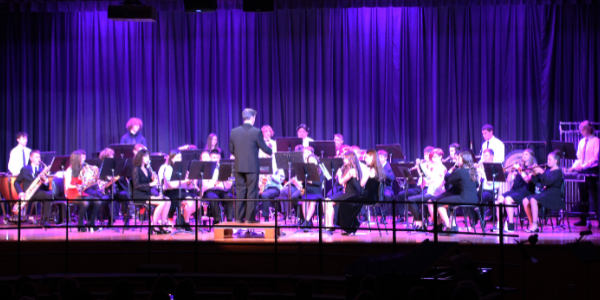The image captures an orchestra performance on a stage, likely at a middle school concert. The conductor, standing on a brown platform, faces a group of young musicians as they look back towards him for guidance. The stage is lit with a blend of purple, pink, and spotlight illumination, creating a vibrant atmosphere. A deep blue curtain forms the backdrop of the stage, with a crowd present but rendered indistinct due to a darkened auditorium. The orchestra is composed of various instruments, including violins, pianos, saxophones, flutes, timpani, and possibly other woodwinds. A railing is visible at the front of the stage, adding a structural element to the scene.